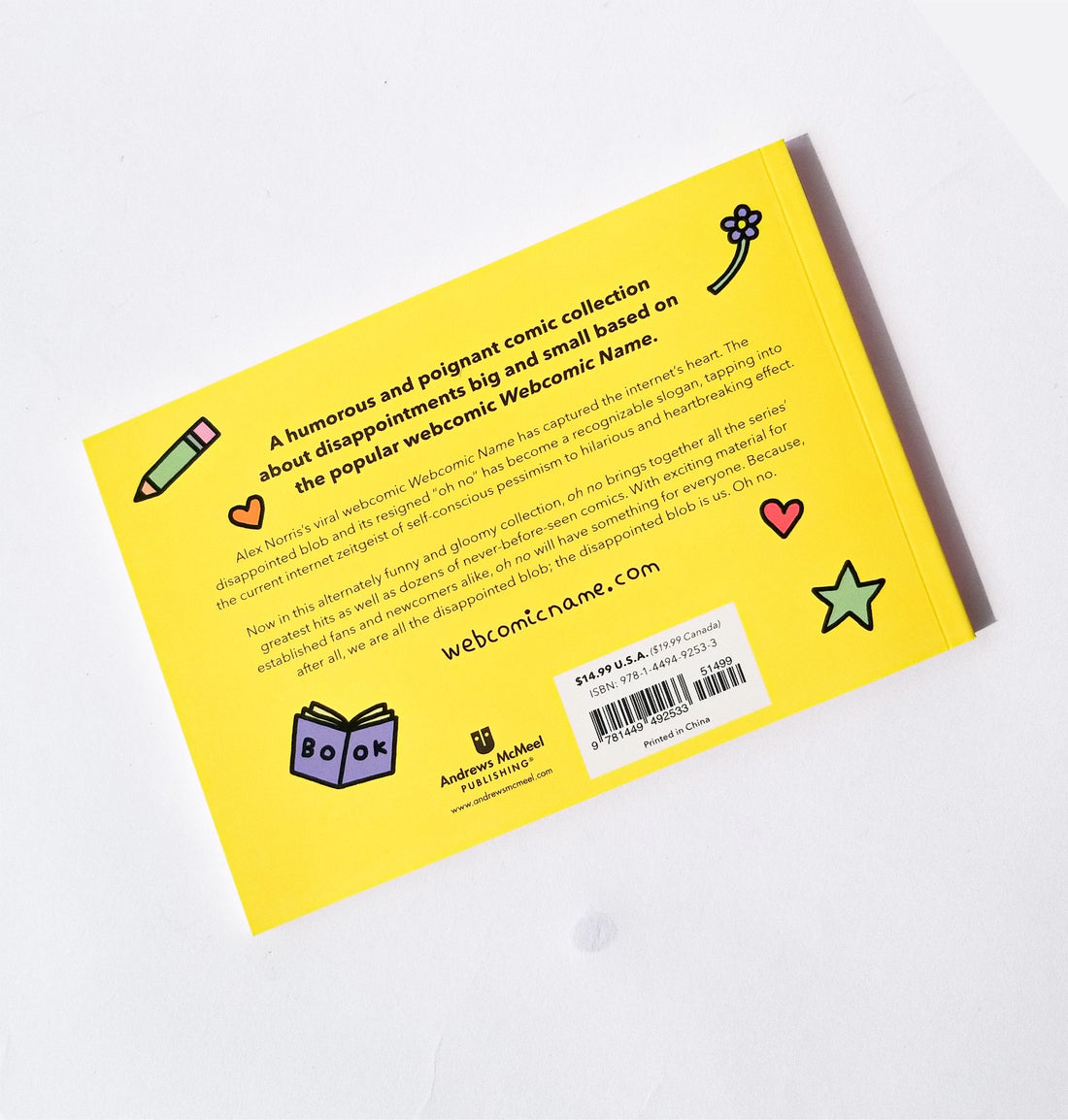This detailed color photograph shows the back cover of a book set against a gray background. The cover is a vibrant yellow adorned with various illustrations in the corners: a cartoon pencil in the upper left, a delicate flower in the upper right, a heart and a star in the lower right, and a cartoon book in the lower left. Above these visuals, bold black text captures attention: "A humorous and poignant comic collection about disappointments, big and small, based on the popular webcomic Webcomic Name." 

Following this, two paragraphs of smaller black text describe the book's content and its origins. The first paragraph reads: "Alex Norris's viral webcomic Webcomic Name has captured the Internet's heart. The heart, the disappointed blob and its resigned 'Oh no!' has become a recognizable slogan, tapping into the current Internet zeitgeist of self-conscious pessimism to hilarious and heartbreaking effect." The second paragraph states: "Now in this alternately funny and gloomy collection, 'Oh no!' brings together all the series' greatest hits as well as dozens of never-before-seen comics. With exciting material for established fans and newcomers alike, 'Oh no!' will have something for everyone. Because, after all, we are all the disappointed blob. The disappointed blob is us. Oh no!"

Also present on the cover are the URL "WebcomicName.com," the logo of the publishing house Andrews McMeel Publishing, and a white price label bearing the text "$14.99" and "Printed in China," along with a UPC barcode.